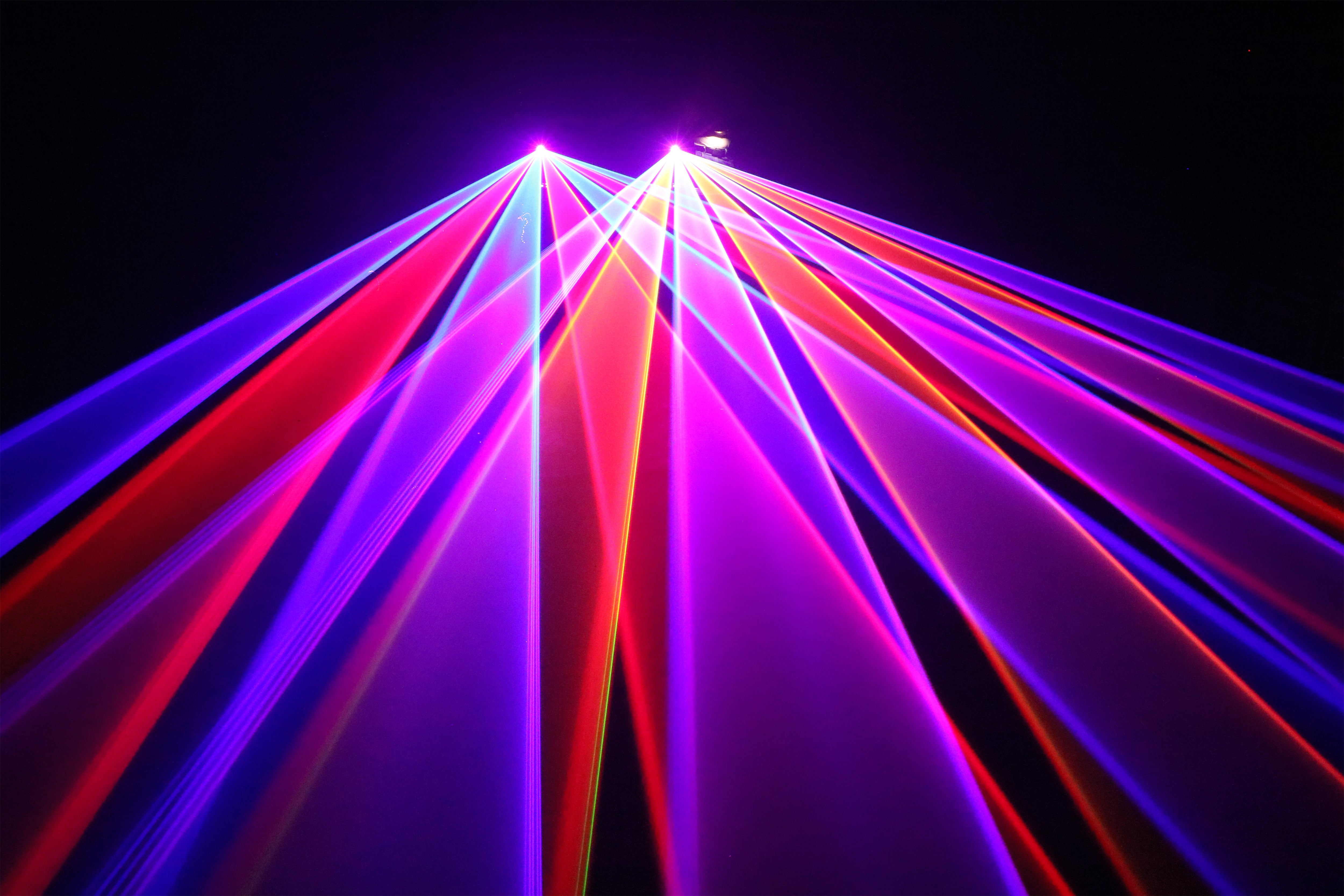The image showcases an abstract, photography-style depiction featuring two distant, circular spotlights mounted on the roof, casting vibrant rays of light in a nightclub or gig setting. The spotlights project numerous strands of light—around seven from each source—creating a mesmerizing display of overlapping colors including pink, purple, red, and hints of blue and orange. These colorful streaks expand and widen as they approach the bottom of the image, resembling a road-like pattern that converges into two vanishing points. The overlapping strands blend in the center to form a kaleidoscope of hues against a stark black background, highlighting the contrast and vividness of the light beams.